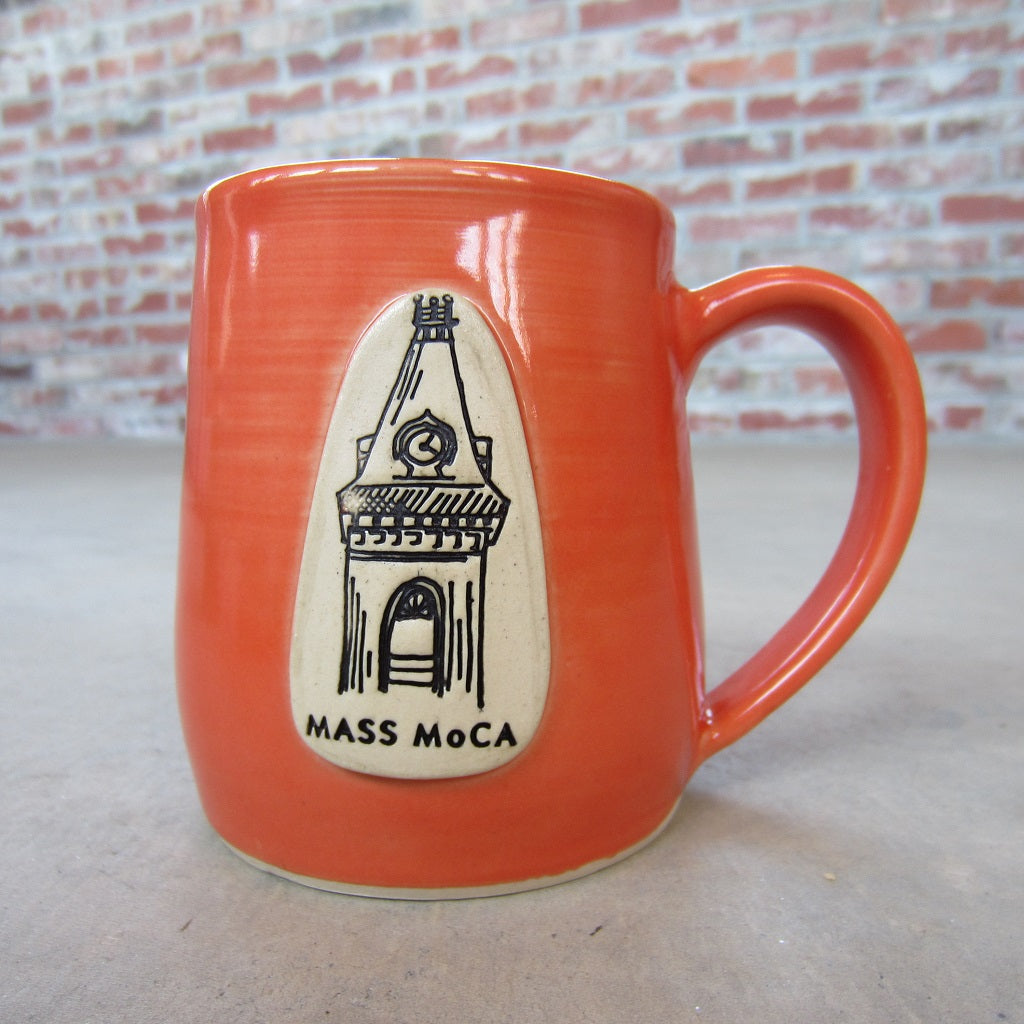The image depicts an aged, spackled brick wall midway up, contrasting with a white floor below. Centrally positioned is a large, flamingo-pinkish orange coffee mug, approximately 16 ounces with a curved handle and a rounded upper lip. The bottom edge of the mug is accented by a white line. Prominently displayed on the mug is a detailed black illustration set within a white oval. The illustration features a castle-like clock tower with a pointed roof, adorned with a clock, a small flat circular surface with railings on top, and a window below the roof. Beneath the illustration, the mug is inscribed with "Mass Mocha" in bold black text.